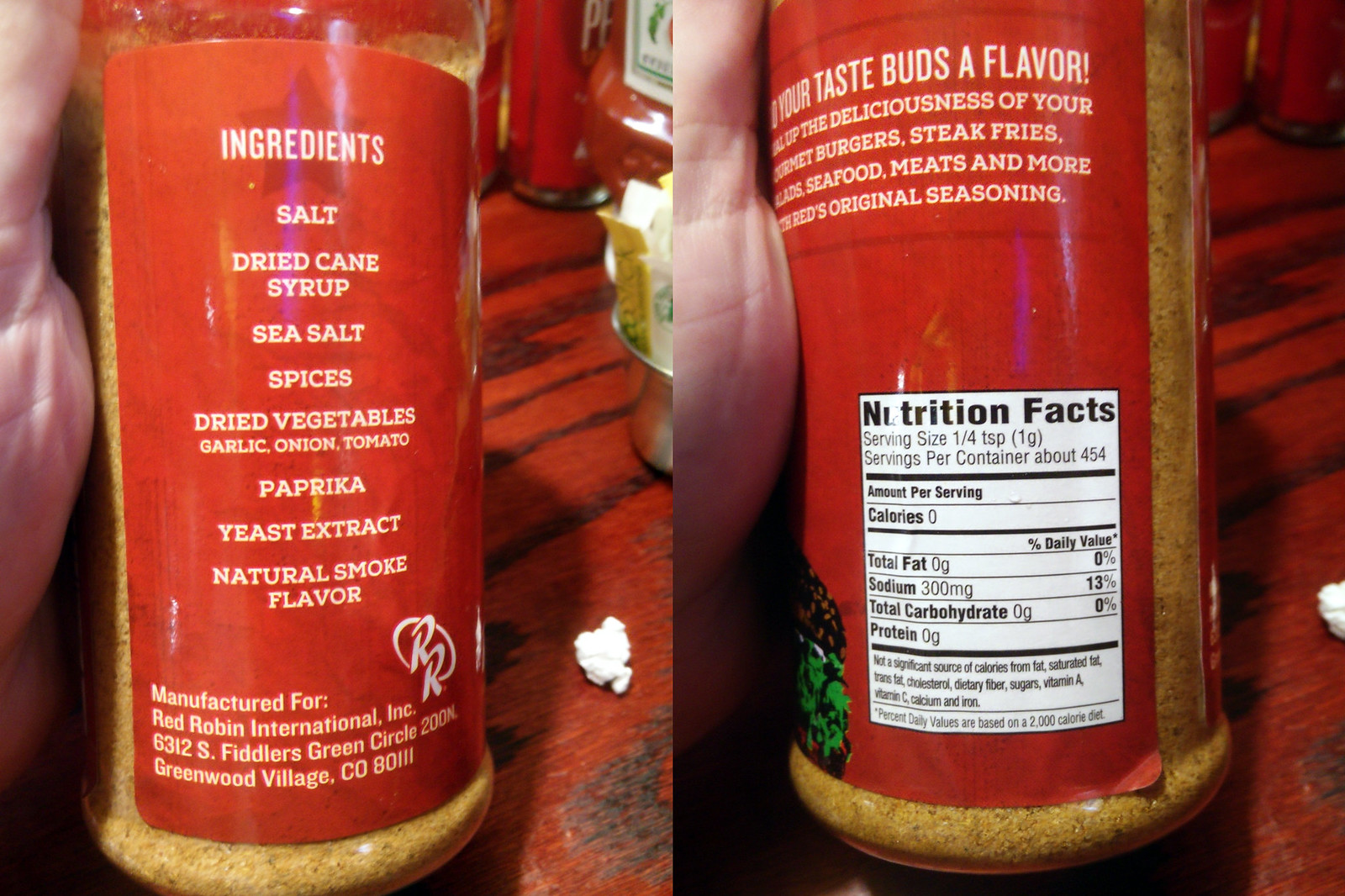The image comprises two side-by-side photographs of the same plastic spice jar. The photograph on the left focuses on a segment of the jar's label, which is a vibrant red rectangle. The topmost part of the label prominently displays the word "Ingredients" in red text. Following that, the listed ingredients are: "Salt," "Dried Cane Syrup," "Sea Salt," "Spices," "Dried Vegetables," "Garlic," "Onion," "Tomato," "Paprika," "Yeast Extract," and "Natural Smoke Flavor." The lower-left corner comprises four lines of text. Through the jar's transparent plastic, the contents of the spice mix are visible, showing a tan-colored blend interspersed with brown dots. The backdrop for this part of the label remains red.

In the photograph on the right, a different section of the same jar's label is shown. Although the top part of the text is cut off, one can make out the partially visible word followed by "TASTE BUDS OF FLAVOR" in bold white uppercase letters. Below this header, there are four more lines of white text. At the bottom-right corner of this section of the label, the square-shaped Nutrition Facts box is noticeable.